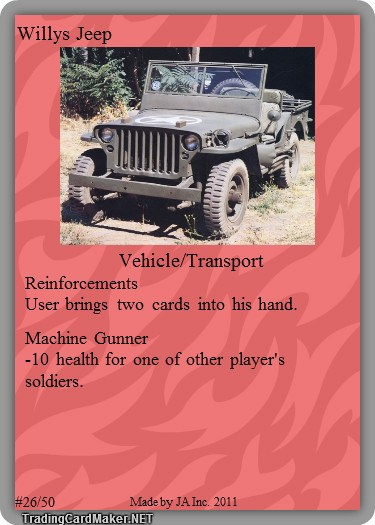The image depicts a roughly conceptual trading card designed for a game. The card has a dark gray border surrounding a red background that features an abstract pattern of curved shapes, which could resemble flames. At the top of the card, "Willie's Jeep" is written in dark text. Below this, there's a color photograph of an old, 1950s-style army jeep, similar to those used in the TV show MASH. The jeep has an olive green body, no roof, and large tread tires, and it is parked on golden grass with plants visible in the background. Beneath the photograph, the following text appears: “Vehicle/Transport” in the center, followed by “Reinforcements: User brings two cards into his hand” aligned on the left. Further down is “Machine gunner: -10 health for one of the player’s soldiers.” At the very bottom, the card indicates “26/50” and the text “tradingcardmaker.net” is inscribed in white within the border. The overall style of the card combines photographic realism with graphic design elements.